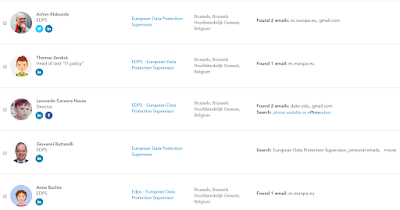This image depicts a grid of five profile pictures, each accompanied by various icons and text. The image is small, making it difficult to discern details clearly. The top row begins with an individual who appears to be male and bald. Next to this profile is a name and two light blue icons. 

Moving to the other profiles, four of them seem to depict males, while one could possibly be female. Three of the images resemble real photographs, and two are more cartoonish avatars. The bottom row, specifically in the middle, features what looks like a child's profile picture. This child's profile is also accompanied by two icons similar to the first profile: a blue and a light blue icon.

All profiles have some form of an icon next to them, with some profiles having two icons, while others have one. The text located next to each profile is too small to be read clearly, though it can be noted that one column of text is highlighted in light blue.